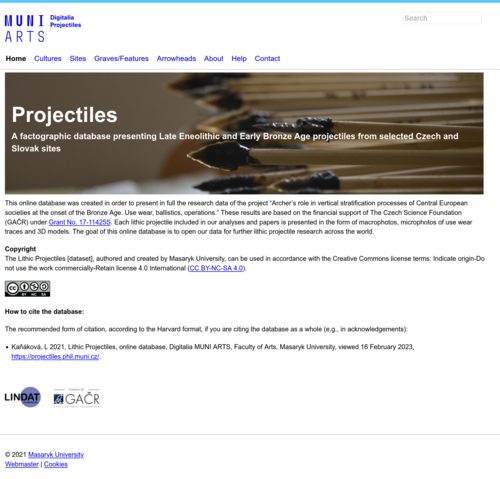Homepage of the MUNI Arts Digital Project: An In-Depth Exploration of Late Eneolithic and Early Bronze Age Projectile Artifacts

This is a detailed view of the homepage of the MUNI Arts Digital Project, focusing on projectiles from the Late Eneolithic and Early Bronze Age periods in Czech and Slovak sites. The site's navigation menu includes tabs for Home, Cultures, Sites, Graves/Features, Arrowheads, About, Help, and Contact. 

Prominently featured is a search box on the right side of the page. The primary focus of this page appears to be a factographic database that presents detailed information and visual representations of projectile artifacts, primarily stone arrowheads, used during these historical periods.

In the main content area, various images of arrowheads are displayed. These artifacts are characterized by their stone composition and bamboo shafts, underscoring their historical significance and craftsmanship. 

Below these visuals, additional text is present but is too small to read. This section includes information on how to cite the database, alongside relevant copyrights and acknowledgments, such as mentions of the LENDAT initiative, GACR, and the year 2021. Text related to copyright information, webmaster details, and cookies policies are also included.

Overall, the MUNI Arts project offers a comprehensive and scholarly resource for the study of ancient projectile artifacts.